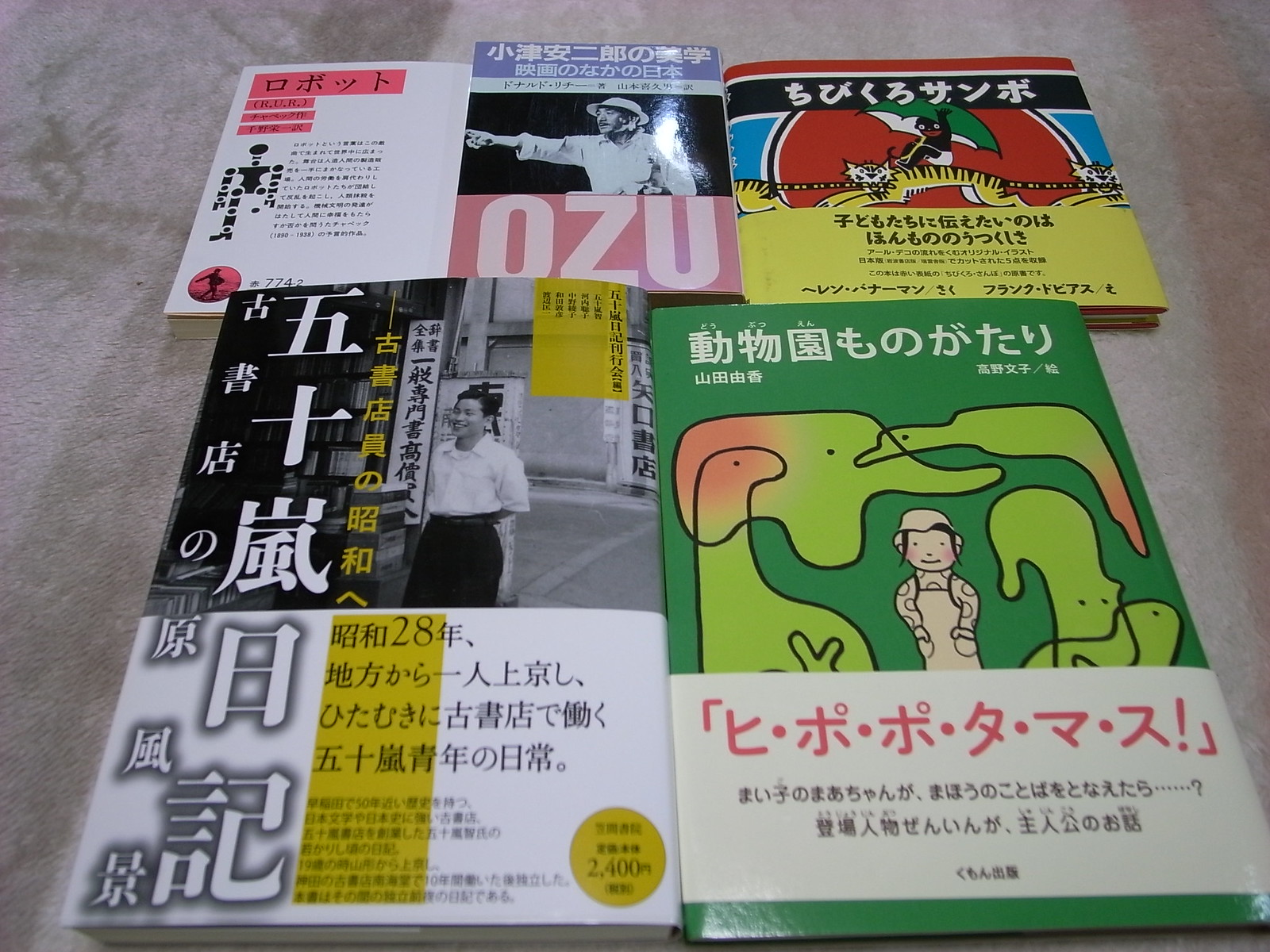The image features an overhead view of five distinct books, all adorned with text in various Asian scripts, laid out neatly on a gray carpet. Two smaller books are positioned at the top, while three larger ones are placed at the bottom. The top-left book is colorful, including figures like a tiger and a monkey with an umbrella. The top-right book, titled "OZU," showcases a performer dressed in a white shirt and a Panama hat. Among the bottom three, the leftmost book in black and white, with yellow shading, depicts a man walking down a road. The middle bottom book has an illustration of a person on a street wearing a white shirt and black skirt. The rightmost book, bright green with light green dinosaurs and red accents, features a cartoon-like figure in the center. This traditional photograph captures the vivid variety and unique details of each publication.